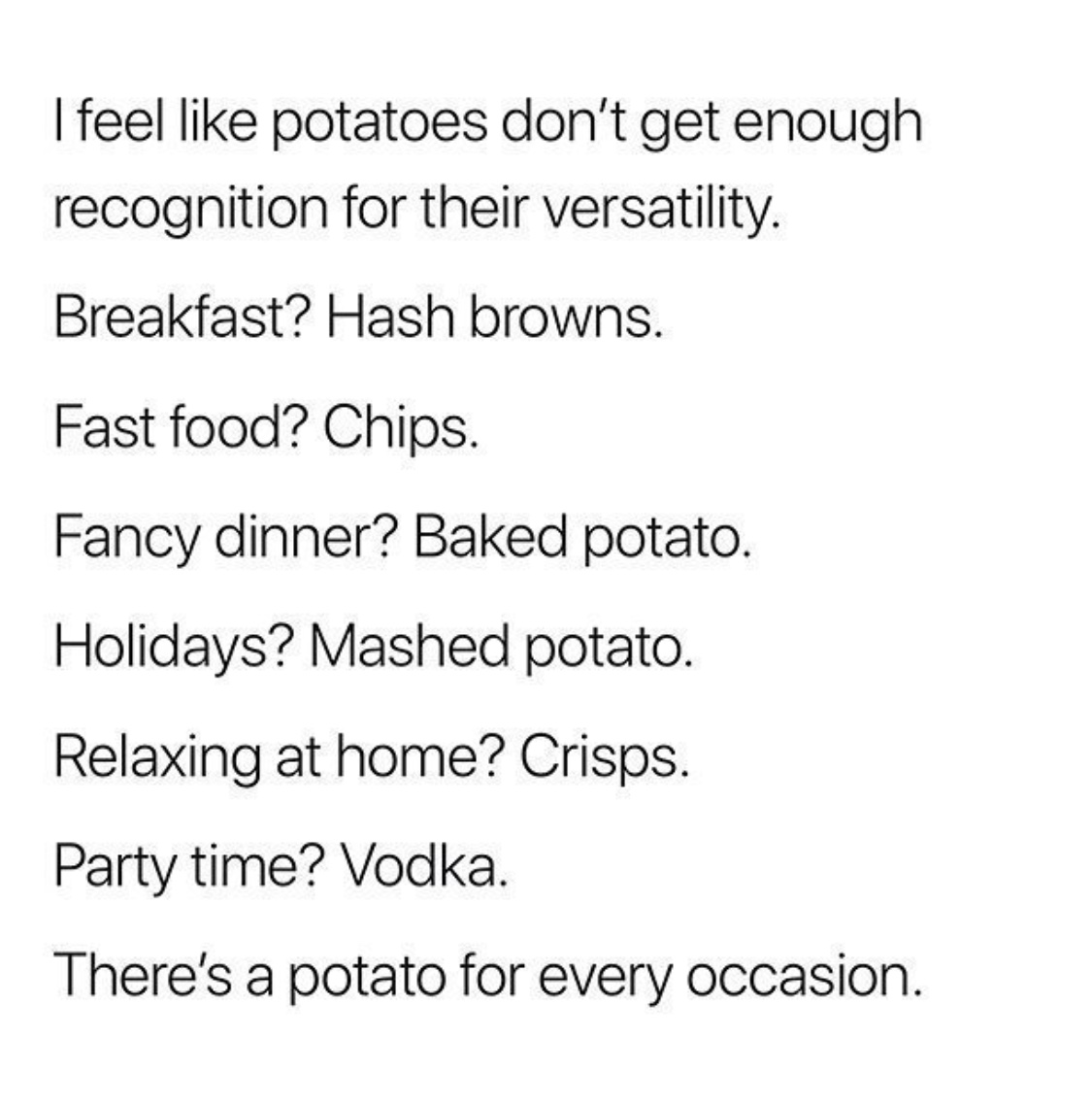The image is a minimalistic meme with black text on a white background. The text spans nine lines and reads: "I feel like potatoes don't get enough recognition for their versatility. Breakfast? Hashbrowns. Fast food? Chips. Fancy dinner? Baked potato. Holidays? Mashed potato. Relaxing at home? Chips. Party time? Vodka. There's a potato for every occasion." This highlights the multifaceted nature of potatoes in various meal contexts, from casual to festive.